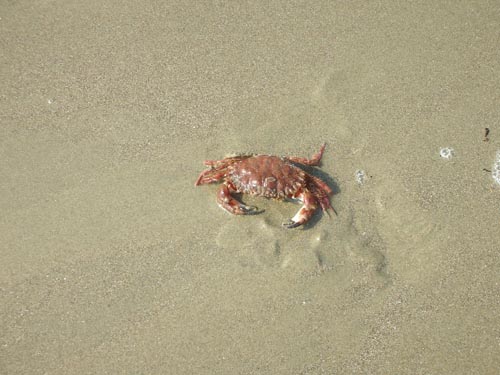This image captures a single red crab, positioned centrally on a wet, sandy beach. The sand is light gray, appearing clean and soft with a slight sheen that suggests recent contact with water. The crab, showcasing a gradient of colors from reddish to tannish brown, with black-tipped pincers, seems to be walking towards the observer. Surrounding the crab, particularly to the right, are clusters of white bubbles peppered sporadically across the moist surface. There are also a few specks of brown debris near these bubbles. The photograph is taken outdoors in the daytime, likely at a coastal location, presenting a minimalist yet detailed scene.